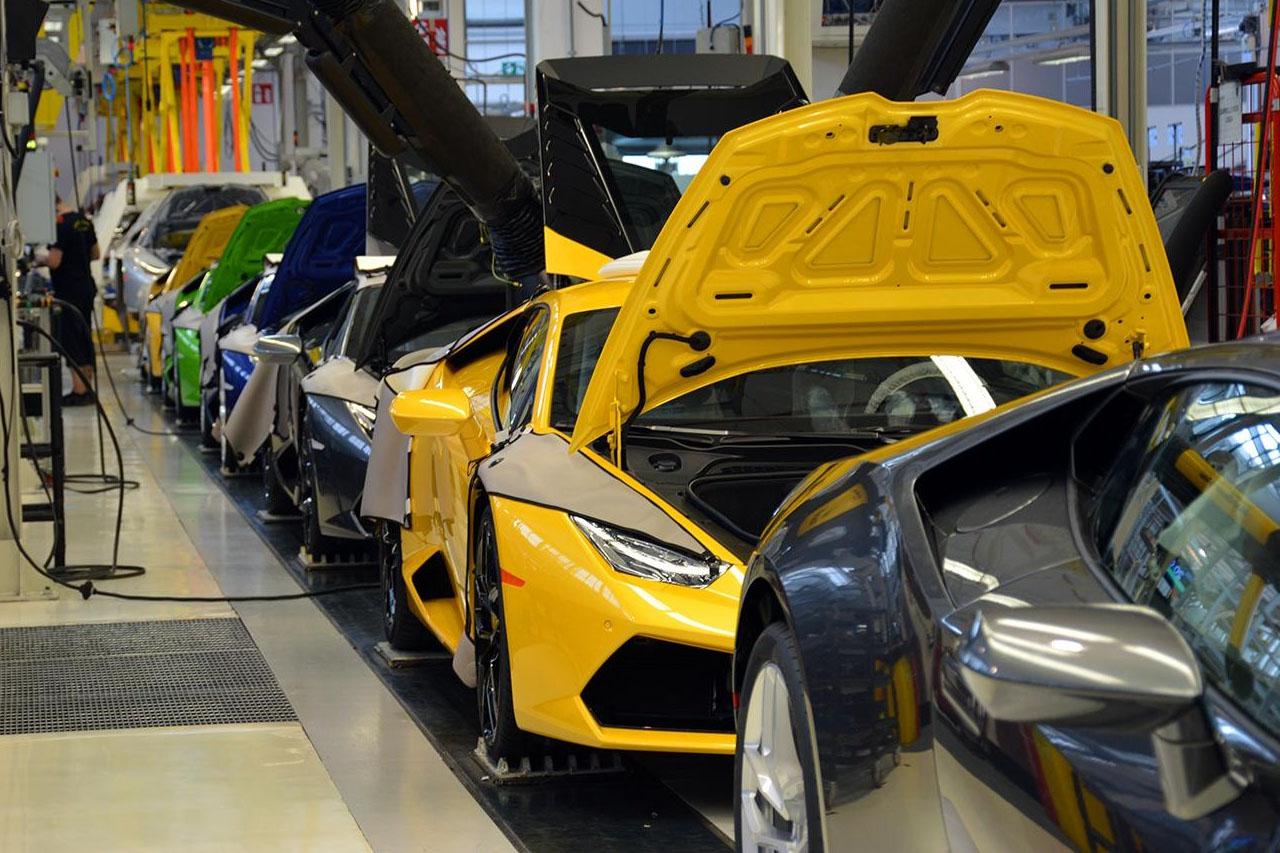The image showcases an assembly line in a sleek, modern car factory where high-end sports cars, resembling Lamborghinis, are meticulously put together. The assembly line stretches from the lower right near the photographer, extending to the upper left, disappearing into the distance. These shiny, brand new cars come in a variety of vibrant colors, emphasizing their luxury and high-quality finishes. A yellow sports car commands the focal point at the center, with its hood open, revealing part of its right front end including the headlights. A series of similarly open-hooded cars line up behind it, displaying their black, silver, blue, lime green, and another yellow hood. The floor is pristine, composed of large, light tan, and cream-colored tiles with a drain visible among them on the left side. A worker, dressed in black shorts and a black t-shirt, can be seen in the upper left corner, diligently attending to the assembly process. The factory is well-lit with bright white ceiling lights and features large windows on the upper right side, allowing natural light to flood the workspace.